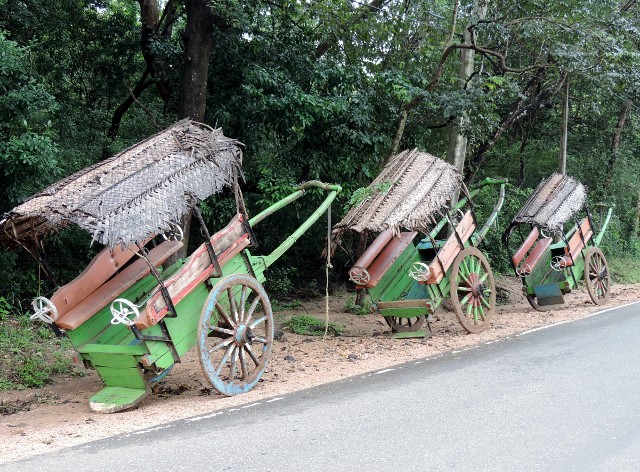The image depicts three wooden carriages, each tipped over and rendered in intricate detail, situated on a sandy dirt area adjacent to a main path. These carriages feature thatched, brown straw roofs attached to two long, bench-like seats, which face each other and are possibly made of wood—one described as salmon-colored. Each carriage's base is composed of green wooden slats with a rounded wooden step at the bottom. The wheels vary in color, including blue, brown, and salmon and green. A distinct, large metal handle, also painted green, extends from the back of each carriage, suggesting they might be horse- or donkey-drawn. The scene is set against a backdrop of lush, dark green trees, grounding the image in a natural, leafy environment.